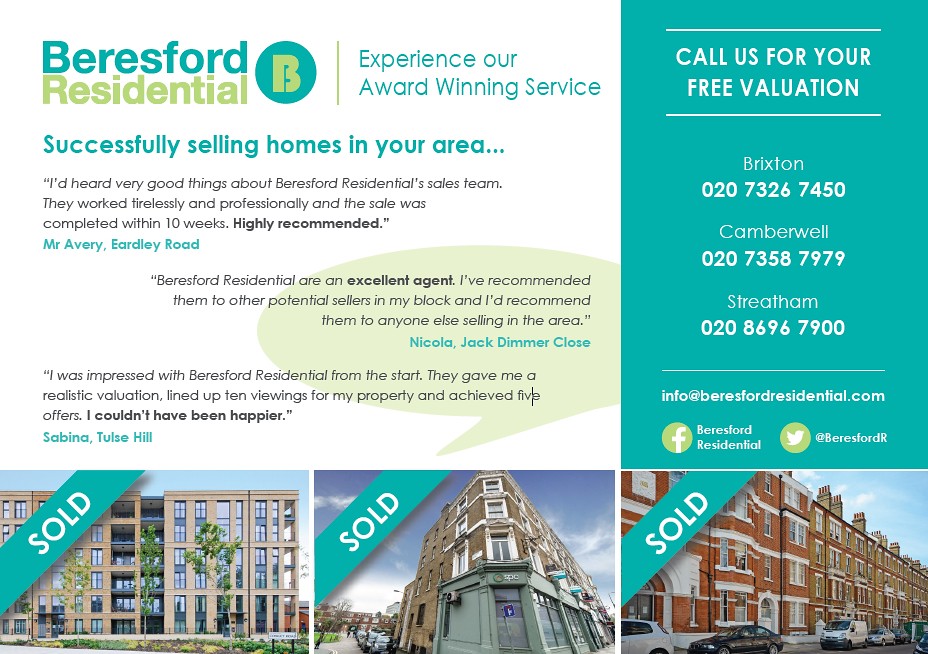This image is a detailed advertisement for Bearsford Residential, a real estate company. The ad is sectioned into five distinct areas. The upper left portion features a white background with light blue writing that reads "Bearsford Residential." The word "Bearsford" is in light blue, while "Residential" is colored gold. Adjacent to this, there is a blue circle with a gold 'B' logo. To its right, the text "Experience our award-winning service, successfully selling homes in your area" is prominently displayed in blue.

Below this, the ad includes three testimonials from satisfied customers, emphasizing the positive experiences of previous clients. 

The lower fourth of the image showcases three square photos of properties that have been sold. These photos depict apartment buildings, the corner of a brick building, and a row of brick houses. Each image has a blue banner with the word "SOLD" written in white, diagonally stretching across the upper left corners.

On the right side of the advertisement, a large blue background contains white print, urging viewers to "Call us for your free evaluation." It lists contact numbers for three locations—Brixton, Camberwell, and Streatham—followed by the website address, "info@bearsfordresidential.com," and social media links for Facebook and Twitter.